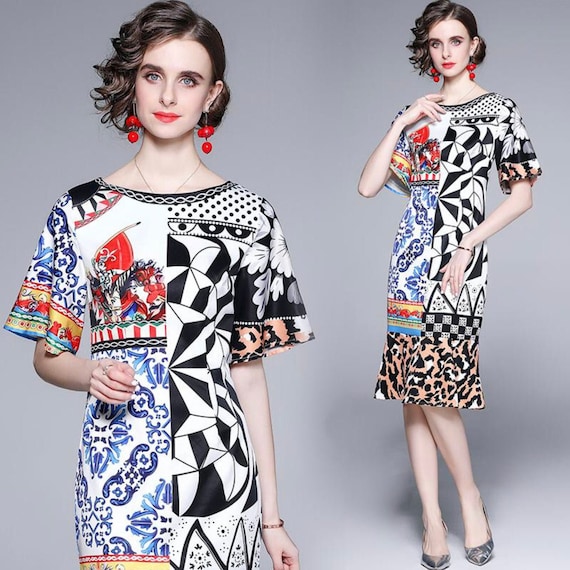The image is a square-shaped photograph featuring a pale-skinned woman with short, almost black hair styled in a ponytail, slightly curled on the left side. The image is composed of two separate photographs of the same woman, wearing the same outfit but taken from different angles. The left photo displays her from the waist up, while the right photo captures her full body. 

In the left image, the woman wears red pearl earrings and sports red lipstick with eye makeup that accentuates her grey-colored eyes. Her outfit is a short-sleeve white dress adorned with multiple different patterns. The right sleeve features black fabric with white floral designs, whereas the left sleeve is white with blue floral patterns. The left chest area depicts knights charging into battle, including a red flag, while the right chest section showcases various black and white geometric patterns.

In the right image, the woman's full outfit is visible, including her black pointed high heel shoes. The lower portion of the dress has abstract blue floral patterns on a white background and a cheetah print at the very bottom. The entire ensemble stands against a plain grey backdrop, highlighting the intricate and colorful designs of the dress as the woman poses elegantly.